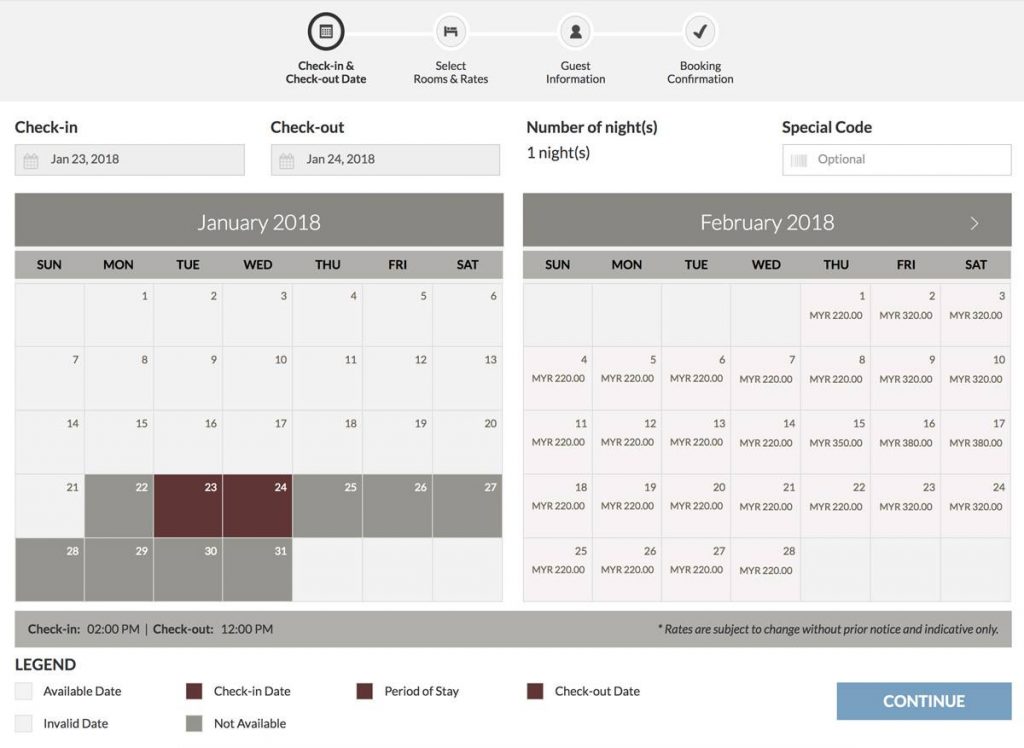"Screenshot of a hotel booking page for an overnight stay on a predominantly white background featuring multiple gray-toned boxes. At the top center, there are four horizontally aligned circles labeled 'Check-in and Check-out Date,' 'Select Rooms and Rates,' 'Guest Information,' and 'Booking Confirmation.' The 'Check-in and Check-out Date' circle is encased in a thick black border, indicating the active step one of four. The user is booking a stay for January 23rd to January 24th, 2018, as shown by the filled-in check-in and check-out dates. The number of nights is specified as one.

On the far right, there's a box for 'Special Code,' where a coupon or discount code can be entered. Central to the page are two monthly calendars for January and February 2018, allowing users to select and view room prices. The dates January 23rd and 24th are highlighted in maroon indicating the selected check-in and check-out dates.

At the bottom of the calendars is a legend explaining the color codes: maroon for check-in/check-out dates, dark gray for unavailable dates, light gray for available dates, etc. The bottom right of the page features a blue 'Continue' button in white text, to proceed with the booking process after date selection."